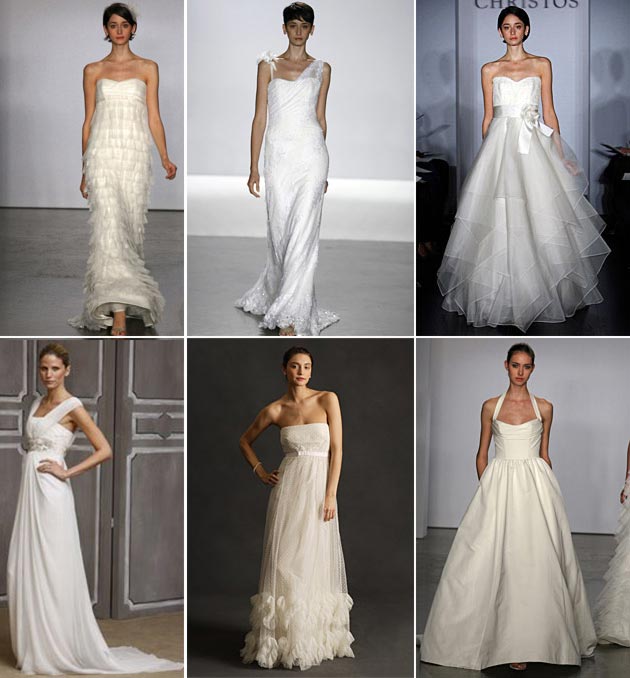This image displays six fashion runway photographs of different models showcasing a variety of wedding dresses. The layout features three dresses on the top row and three on the bottom row. Each dress is unique in style yet all share a common bridal theme in pure white. 

- The top left dress is sleeveless with a frilly, fluffy design reminiscent of a flapper dress, exuding an elegant vintage flair.
- In the top middle, a floor-length gown stands out with its pure white hue, featuring asymmetric straps — one shoulder adorned with a bow and the other an off-the-shoulder lace strap.
- The top right dress opts for a more whimsical Cinderella-like aesthetic, being strapless and accentuated by a sizeable bow at the midriff.

On the bottom row:
- The bottom left gown has lace straps and no sleeves, complemented by a belt situated just below the bust.
- The bottom middle dress, fashioned from lace material, flares out slightly at the bottom and sports a delicate skinny belt below the midriff, all while being strapless.
- Lastly, the bottom right dress adds to the Cinderella charm with its poofy silhouette, featuring a halter strap around the neck, enhancing its fairytale-like presence.

These photos, likely taken during a designer runway event, include visible audience hands and partial text indicating the brand, possibly "Christos", in the background of at least one of the images.